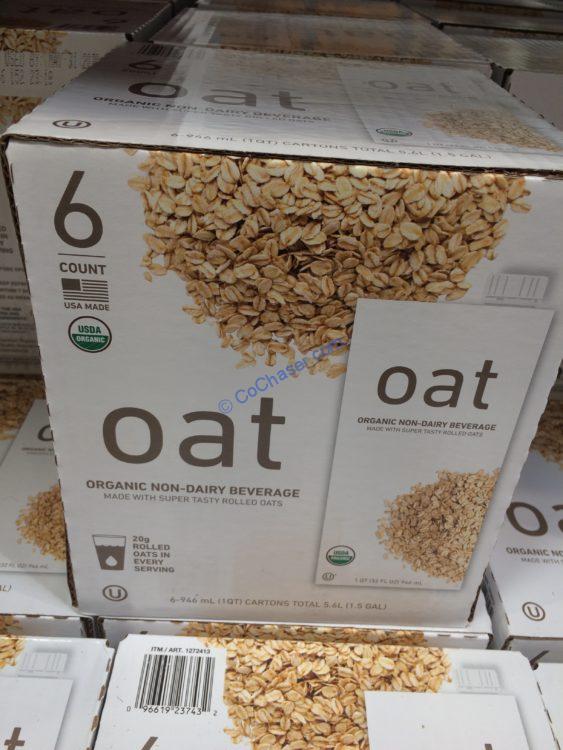The image features multiple branded cardboard containers of oat-based beverages, with one container prominently displayed and fully visible while others are partially stacked around it. The main container has a white background with images of brown oats spread out, resembling them laid on a table. Centered on the container is the word "OATS" in grayish lettering. Below this, the text reads "Organic Non-Dairy Beverage Made With Super Tasty Rolled Oats." 

In the upper left corner, it states "6 Count" with a USA flag underneath, indicating that it is USA made. Below the flag, there's a USDA Organic stamp. On the bottom left of the container, it mentions "20 Grams Rolled Oats in Every Serving." To the right side of the container, there are additional images of oats along with repeated information about the organic non-dairy beverage. The layout prominently highlights the product's organic and wholesome attributes, emphasizing its key selling points in a visually cohesive manner.